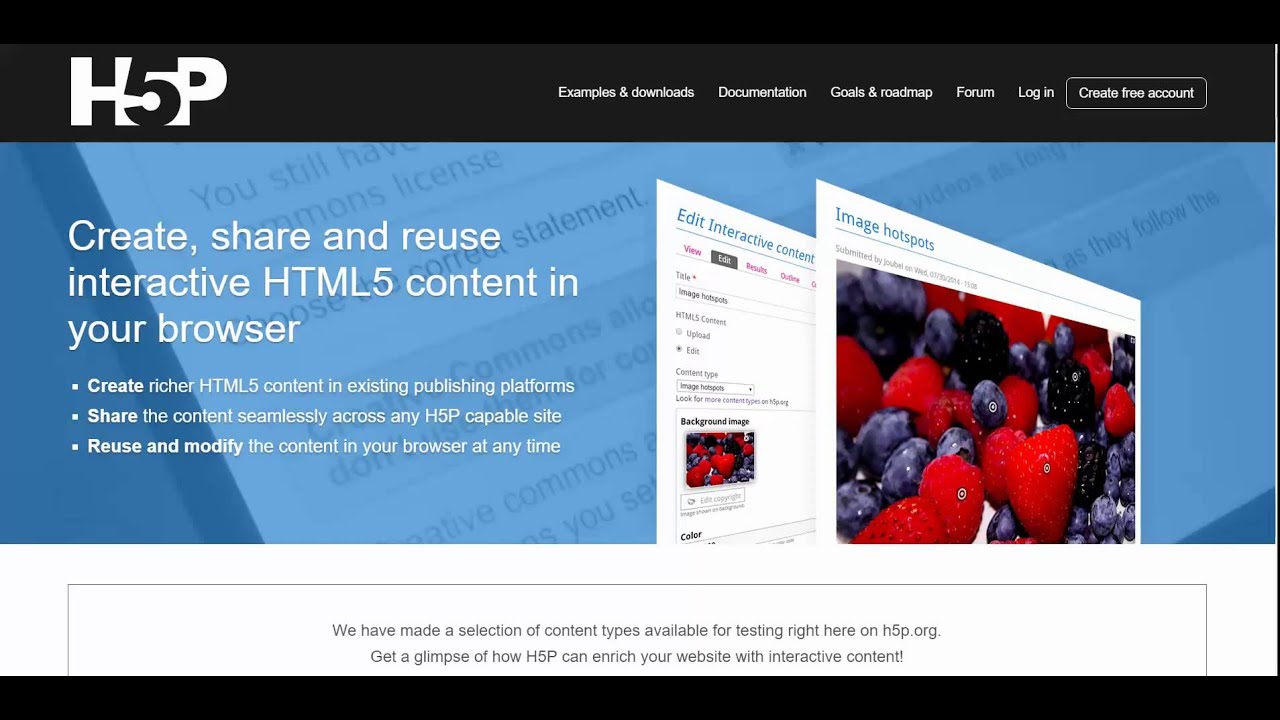The image is a horizontally oriented rectangle with the longer side extending from left to right. Black borders frame the image on both the top and bottom edges. Just below the black border at the top, a dark gray border appears. On the left side of this gray border, the acronym "HP" is prominently displayed in white text, followed by a black numeral "5" situated in the center.

Midway through this gray border, there are several clickable labels in white text: "Example and Downloads," "Documentation," "Goals and Roadmap," "Forum," "Login," and a white-outlined box labeled "Create Free Account."

Below the gray border, the background transitions to an image resembling a computer screen, displaying more text in white. On the left side of this main section, the text reads: "Create, Share and Reuse Interactive HTML5 Content in Your Browser. Create richer HTML5 content in existing publishing platforms. Share the content seamlessly across any H5P-capable site. Reuse and modify the content in your browser at any time."

The overall composition suggests a user interface for a web platform or software related to creating and sharing HTML5 content, with a focus on interactivity and ease of use.